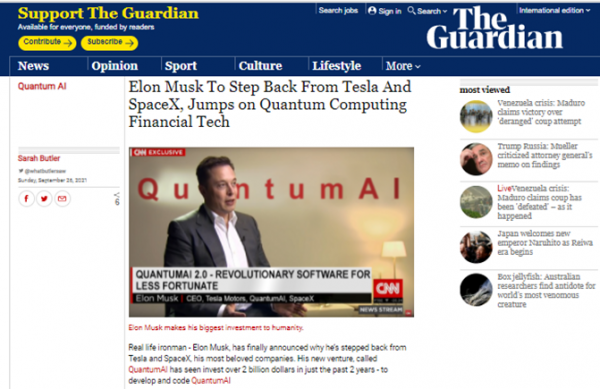The image features a prominent header with a dark blue background. On the top left, bold yellow text in a Times New Roman or Georgia font reads "Support the Guardian." Below this, white text states, "Available for everyone, funded by readers." There are two yellow oval-shaped icons beneath: the first reads "Contribute" with a right-pointing arrow, and the second reads "Subscribe" also with a right-pointing arrow.

On the far right, white text spells out "The Guardian," with "The" above "Guardian." Adjacent to this are several menu options, each bordered by a thin white line: "News," "Opinion," "Sports," "Culture," "Lifestyle," and "More," with "More" featuring a downward-pointing arrow indicating additional options.

A headline in bold black text reads, "Elon Musk to step back from Tesla and SpaceX, jumps on quantum computing financial tech." Below this, an image of Elon Musk is displayed. He is wearing a dark suit coat, and a CNN news ticker below him states, "Quantum: 2.0 - Revolutionary software for less fortunate." A black strip at the bottom is present, though its text is illegible.

To the left, a white bar features red text at the top that reads "Quantum AI." Below this, a thick light gray divider includes the red text "Sarah Butler," indicating the author.

On the right side of the image, a "Most Viewed Headlines" section is visible. Each headline is accompanied by a circular icon featuring an image relevant to the headline.